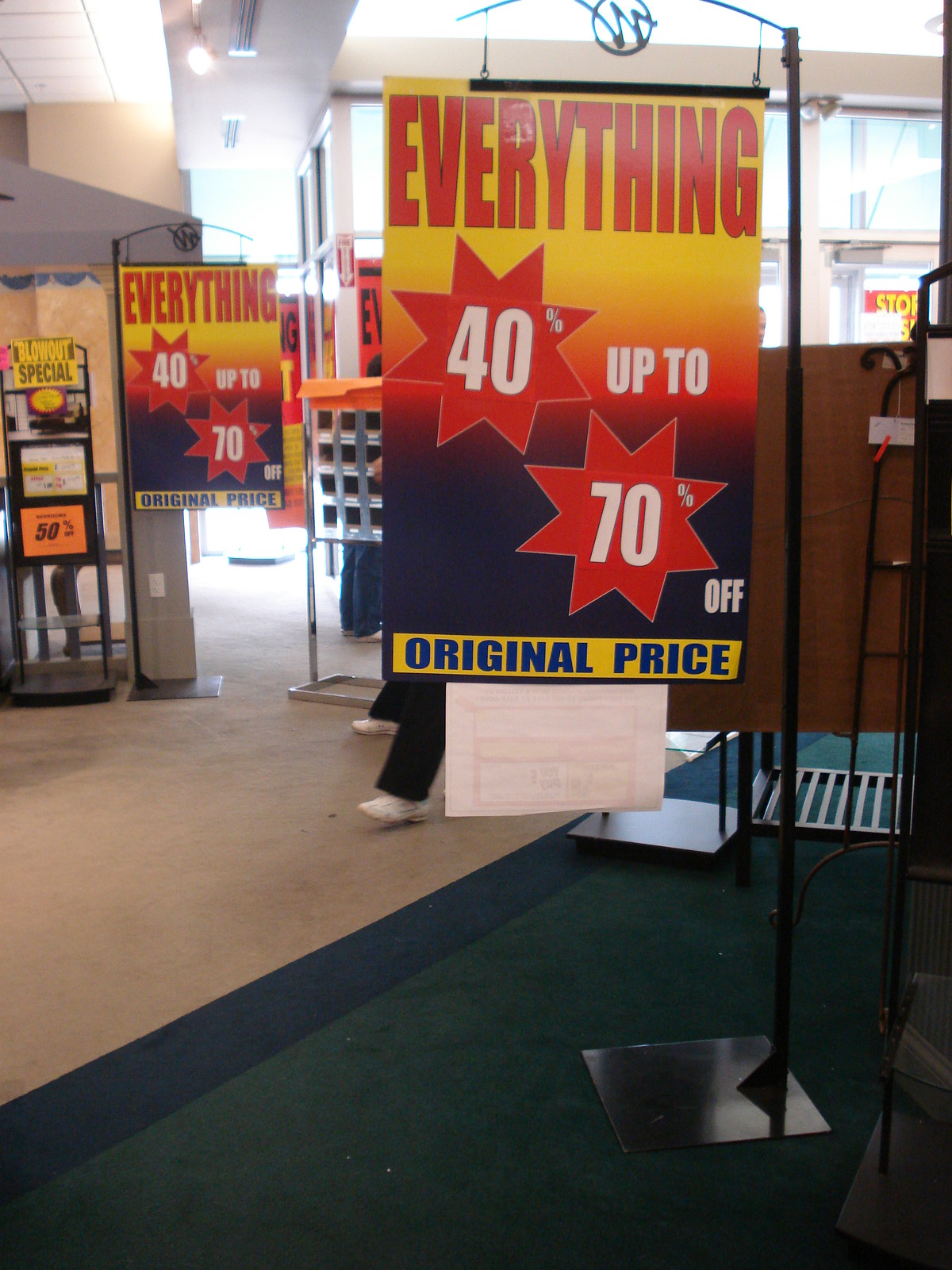This crystal-clear photograph captures the interior of a retail store with remarkable detail. In the foreground, two identical promotional signs are prominently displayed on black metal poles. The signs feature bold red headers with geometric patterns, announcing in white font, "Everything" followed by the striking offer of "40 to 70% off." Below this, a gold rectangle with navy blue lettering indicates "Original Price." The store's floor displays a blend of tan tiles and sections of black and green carpet. Overhead lighting casts an even illumination throughout the space. In the background, automatic white doors are visible, hinting at the store's entrance or exit area. Partially obscured behind one of the signs, a person can be seen, identifiable only by their white shoes and dark-colored pants. The ceiling, in part, also makes a subtle appearance in the top section of the image.